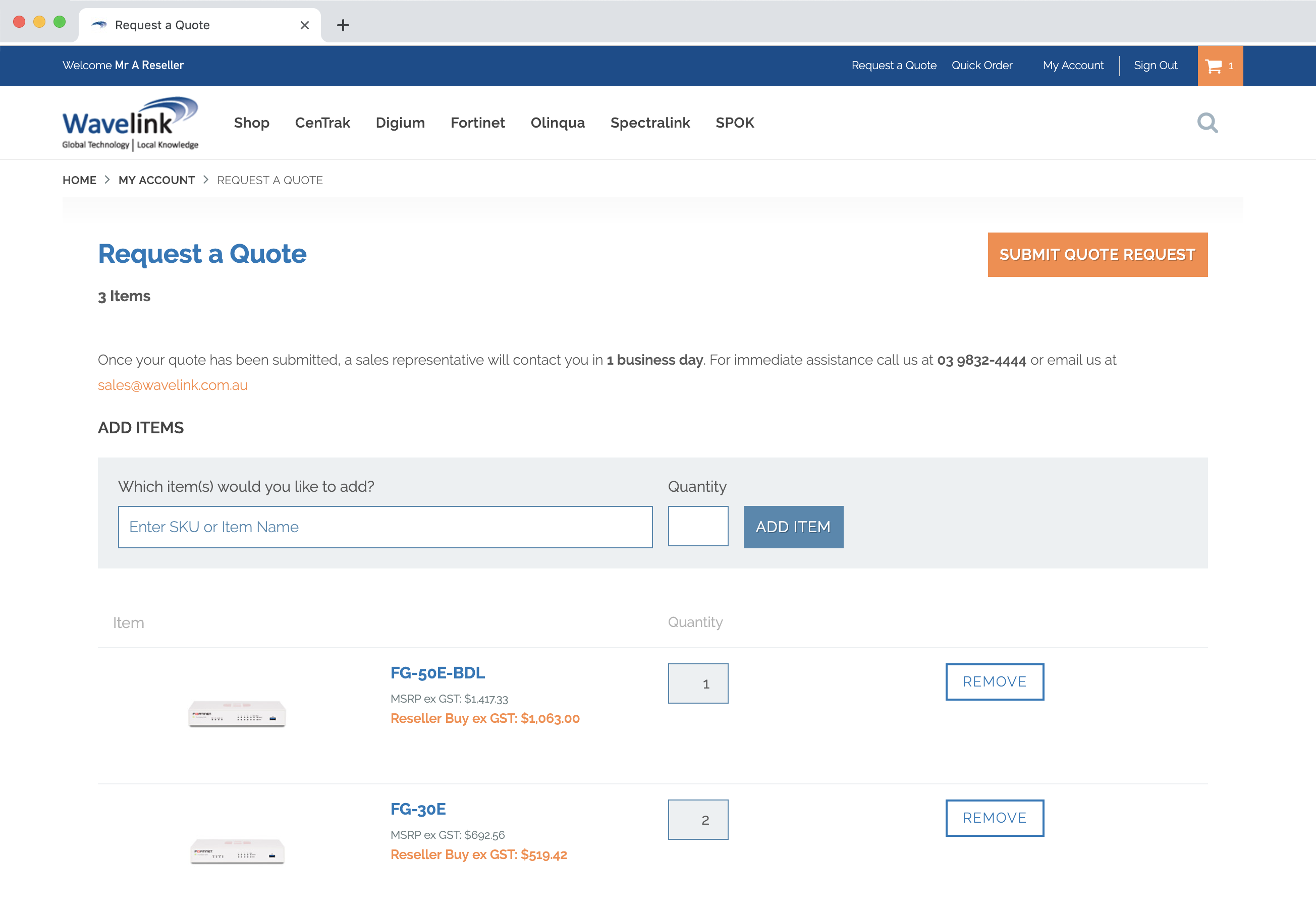An image displays a detailed request form for quotes. At the top, the phrase "Request a Quote" is prominently highlighted in blue letters. Adjacent to this, there's an orange button labeled "Submit Quote Request". Directly below "Request a Quote", it indicates "3 items". A note clarifies that upon submitting the quote request, a sales representative will contact the requester within one business day. Immediate assistance is accessible by calling 0832-4444 or emailing sales@wavelink.com.au.

Beneath this section, in bold black capital letters, the word "ADD ITEMS" is displayed. Under it, there is a light purple box starting with a prompt, "Which item would you like to add?". Below, a text box labeled "Enter SKU or item name" is available for entering item details. Adjacent to it on the right is a smaller textbox with the instruction "Quantity" above it. Further to the right, a blue button marked "Add Item" is positioned. 

In the lower section of the image, there is an item listed: "Item FG-50E-BDL" with a quantity of "1" and an accompanying button labeled "Remove" for deleting the item from the list.